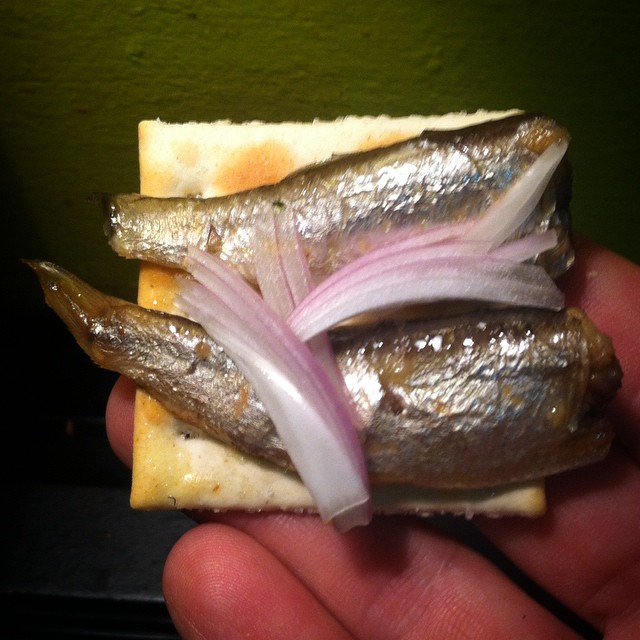A right hand is holding a cracker topped with what appears to be sardines and finely chopped raw onions. The fingers, specifically the pinky and ring finger, are visible as they grasp the cracker. The background of the image is a solid black square, providing stark contrast that highlights the texture and colors of the cracker's toppings.